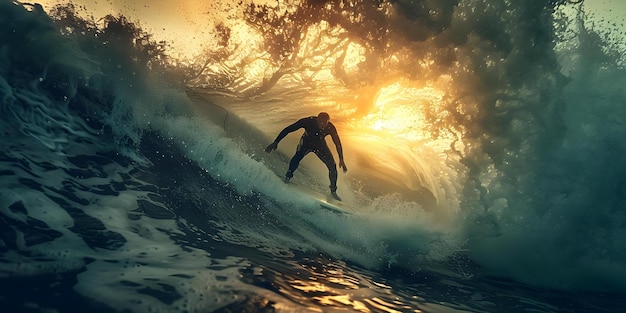In the image, a surfer in a black wetsuit is captured in a striking moment as he rides a colossal wave. The wave, immense and dramatic, cascades from the top left to the bottom right, swirling with shades of purple, dark blue, and white foam. The surfer, appearing almost minuscule in comparison to the gigantic wave, is crouched on his surfboard, balancing expertly amidst the turbulent water. The wave arches powerfully over him, with a section of the sky visible through the translucent water, illuminated by the glow of a golden yellow sun. The upper right of the sky exhibits a gradient of orange, blending into a greenish-blue tint, while the sunlight adds a splash of bright white and yellow to the scene. The overall composition highlights the raw power of nature and the thrilling adventure of surfing, enhanced by the water's dark, almost surreal coloring and the breathtaking action of the moment.